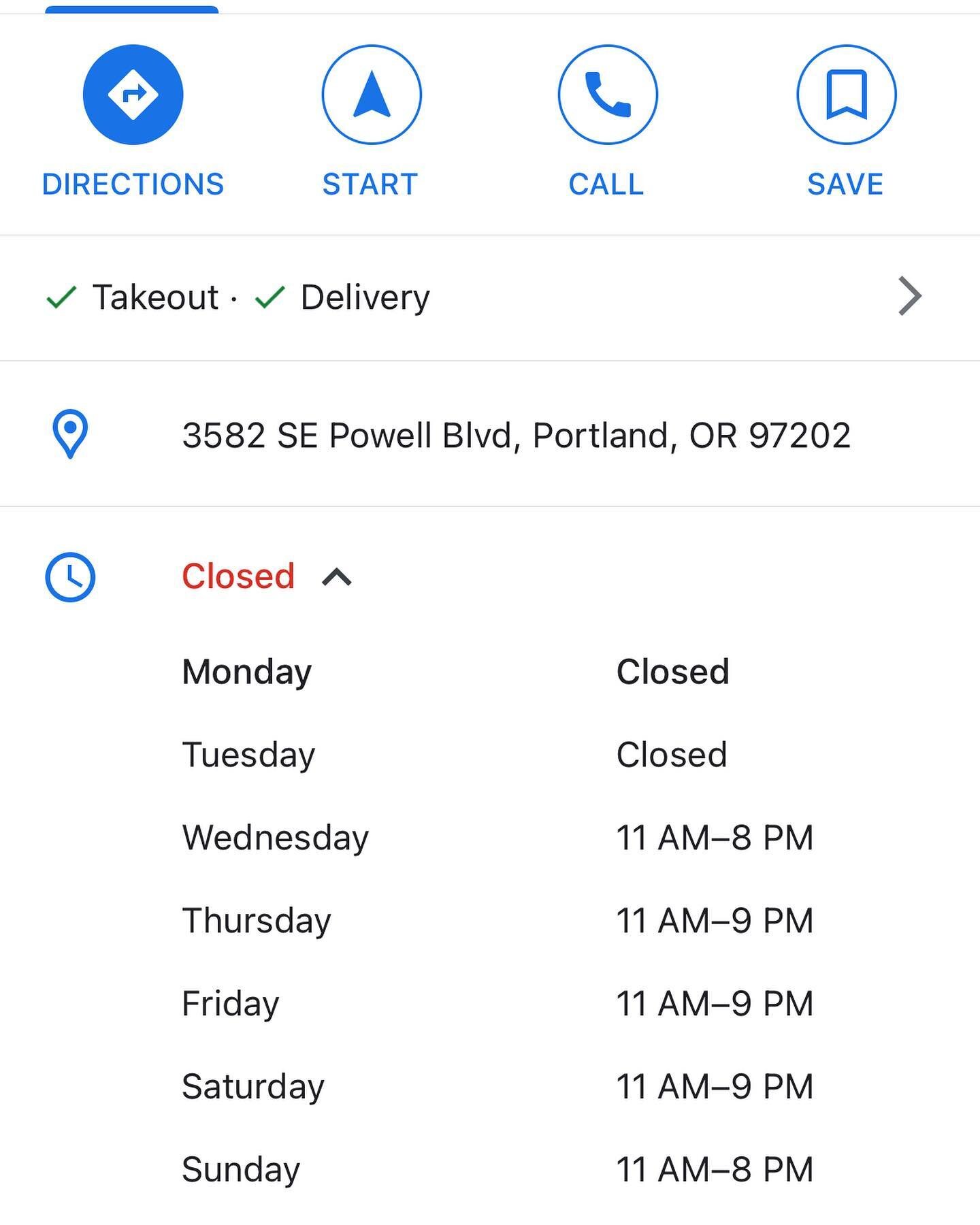This is a detailed image capturing essential Google information about an unspecified restaurant, presented on a white background with black text. At the top of the screenshot, there are four horizontally arranged options: "Directions," "Start," "Call," and "Save." These options allow users to get directions to the restaurant, start navigation, call the restaurant, or save it to their favorites for future reference.

Below these options, on the left center of the screen, the words "Takeout" and "Delivery" appear with green check marks beside them, indicating that the restaurant offers both services. The restaurant's address, listed below this, is 3582 Southeast Powell Boulevard, Portland, Oregon 97202.

The operating hours of the restaurant are displayed underneath the address. At the top, the word "Closed" is prominently shown in red text, indicating that the restaurant is currently not open. The weekly schedule follows in seven rows, detailing the hours of operation for each day. The restaurant is closed on both Monday and Tuesday. From Wednesday to Sunday, different hours are noted:
- Wednesday and Sunday: 11 AM - 8 PM
- Thursday, Friday, and Saturday: 11 AM - 9 PM

Next to the address on the left-hand side of the screen, there is a small blue dot icon indicating the location of the restaurant. Adjacent to the "Closed" status at the bottom half of the screen, there is also a small blue clock icon, suggesting that users can check the operating hours of the restaurant.

This comprehensive snapshot provides all the necessary details a potential customer might need, from the address and hours of operation to service availability and navigation options.